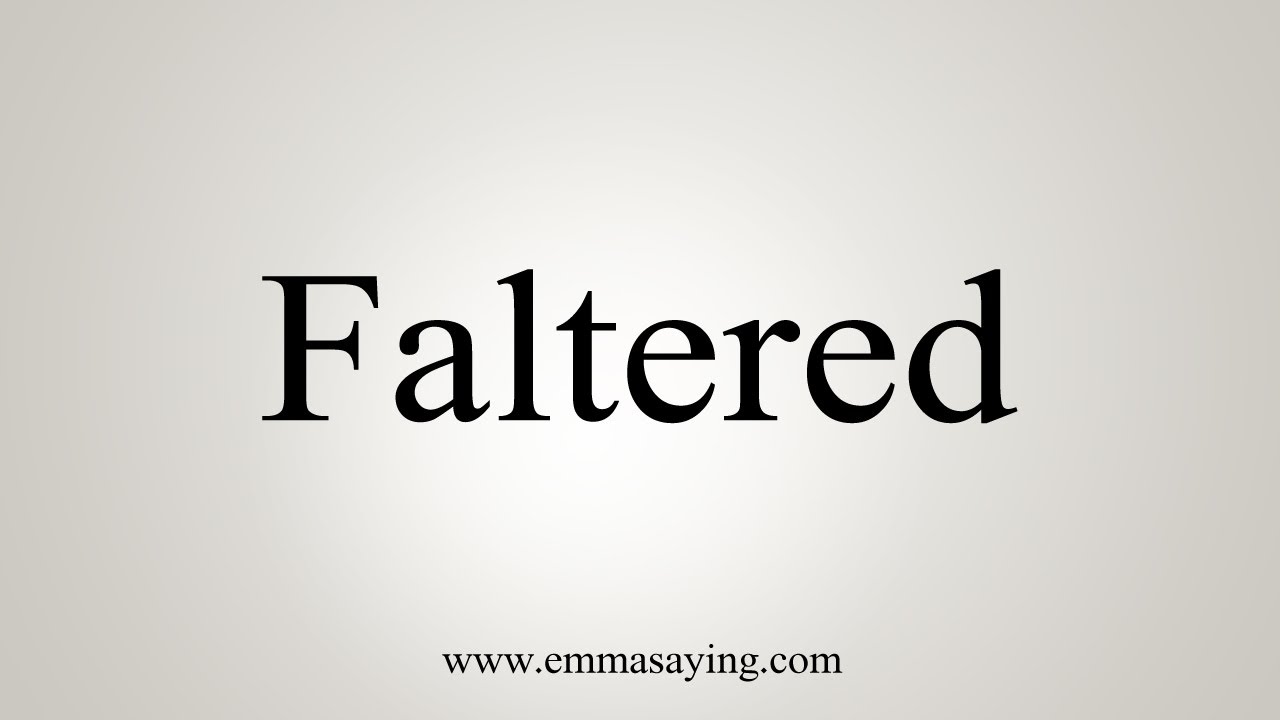The image is a horizontally-oriented rectangle with a very light gray background. In the center of this light gray space, in large black text, the word "Faltered" is prominently displayed, with the "F" being capitalized and the remaining letters in lowercase. The text is large and positioned centrally, creating a significant amount of empty space around it. At the very bottom of the image, also centered but in much smaller black text, the web address "www.emmasaying.com" is written in all lowercase letters. The overall design of the image is minimalistic, featuring only the light gray background and black text, and it appears to be an advertisement of some sort, likely directing viewers to visit the mentioned website. The rectangular shape of the image is approximately 1.5 to 1.75 times wider than it is tall.